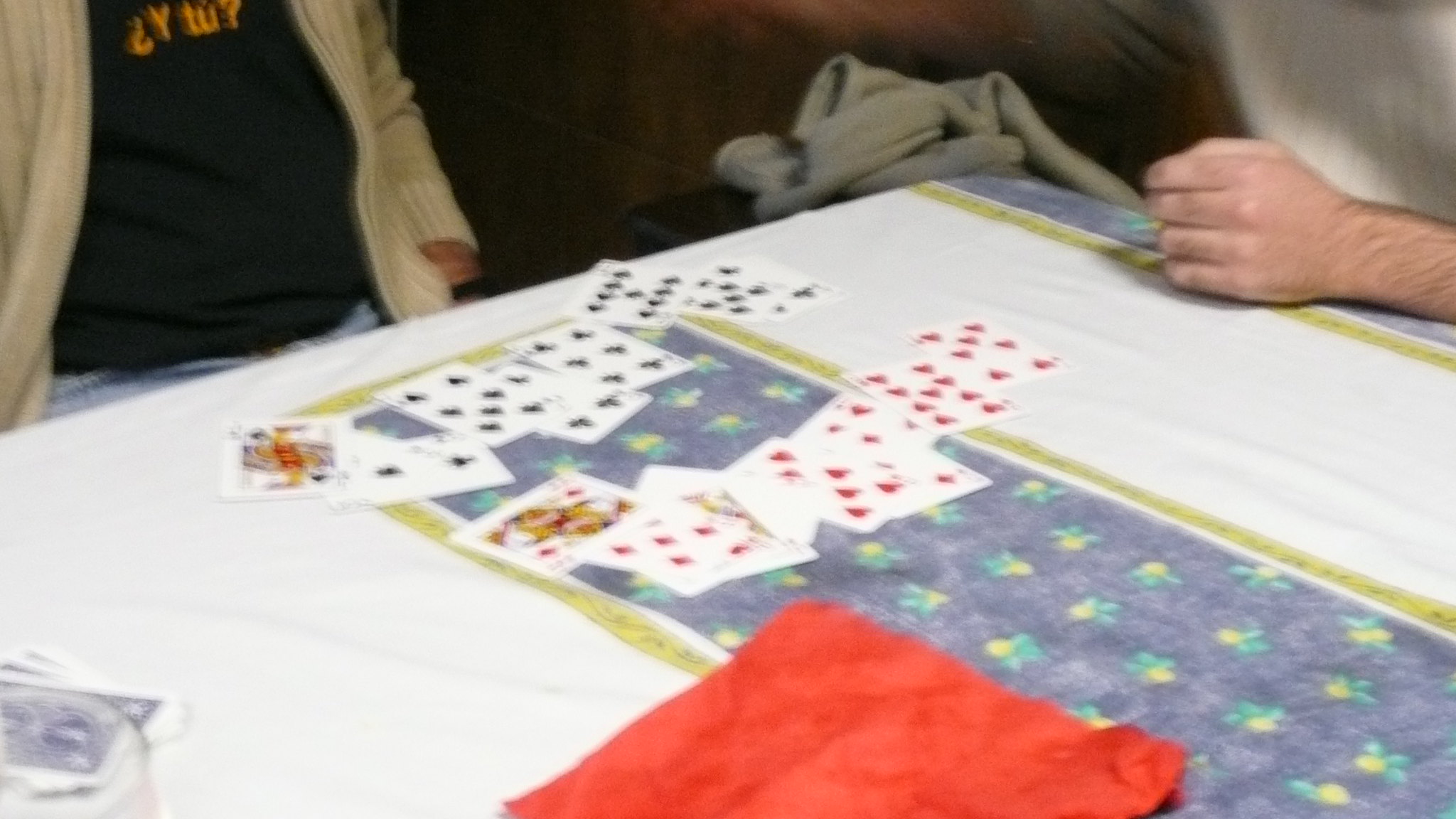This vertical rectangular image captures an engaging scene of two people playing cards at a white table. In the lower left corner, a neatly stacked deck of cards is visible beside a vibrant red napkin positioned at the bottom of the frame. At the center of the table, a blue image of an unknown object draws attention amidst the layout of cards. The cards are methodically arranged with the top row consisting entirely of hearts and the bottom row, spades. To the right side of the image, a man's left hand rests gently on the table surface. On the left side, a partially visible person is seated, donning a black shirt layered under a white sweater, with their left hand casually tucked into their pocket. Both individuals are engrossed in their card game, contributing to the scene’s lively yet focused atmosphere.